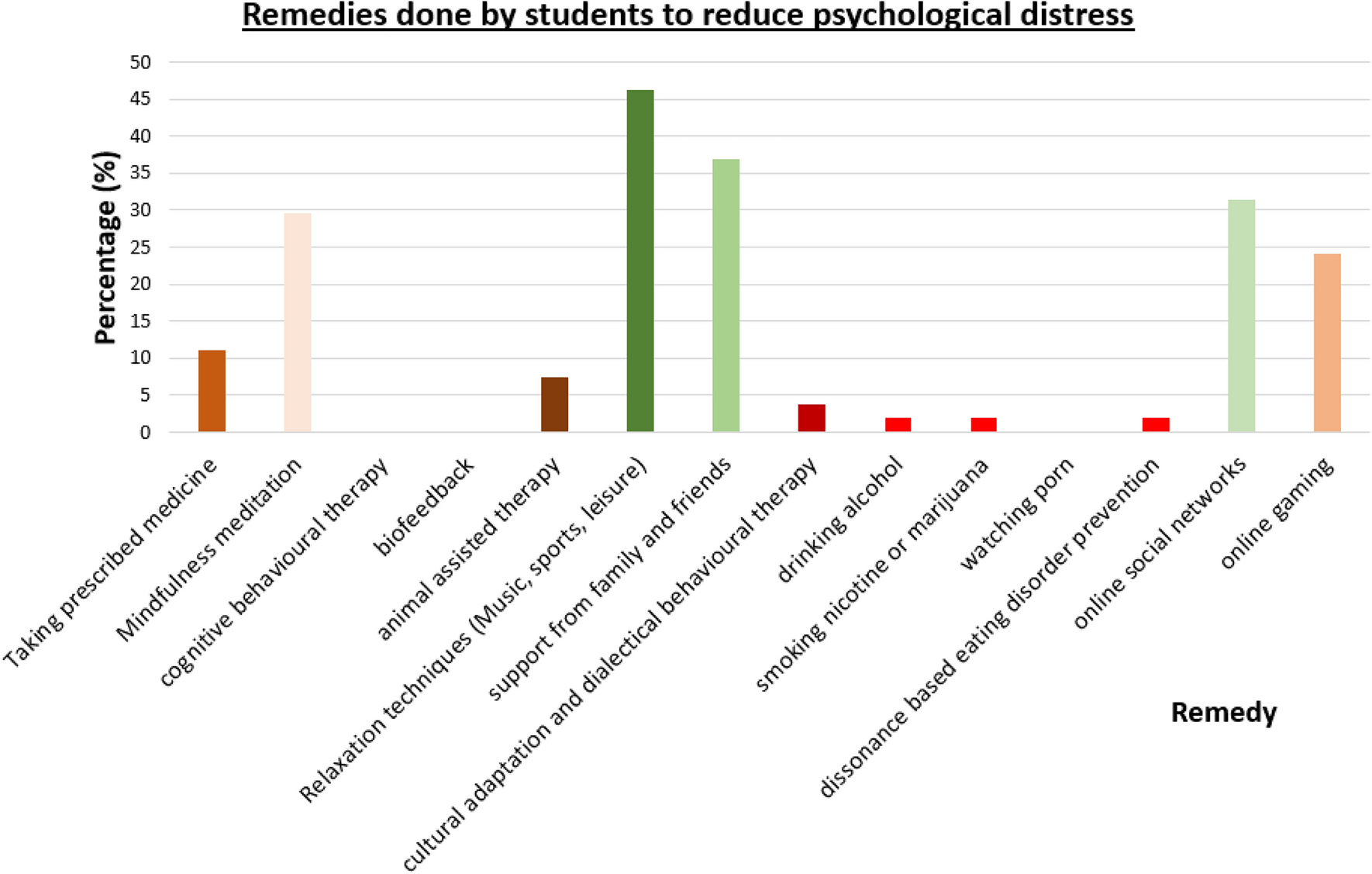The image depicts a detailed bar graph showcasing various remedies employed by students, likely college or high school students, to reduce psychological distress. The y-axis represents the percentage, ranging from 0% to 50% in increments of five, while the x-axis lists various remedies. The highest percentage at over 45% includes relaxation techniques, music, sports, and other leisure activities. Support from family and friends follows closely at around 37%. Mindfulness meditation and online social networks each account for just over 30%. Online gaming is utilized by nearly 25% of students. Other remedies such as taking prescription medicine (10%), animal-assisted therapy (7%), cultural adaptation, drinking alcohol (both around 3%), and smoking (3%) are also noted. Cognitive behavioral therapy (CBT), biofeedback, and watching porn do not register significant usage. The graph is titled "Remedies Done by Students to Reduce Psychological Stress."